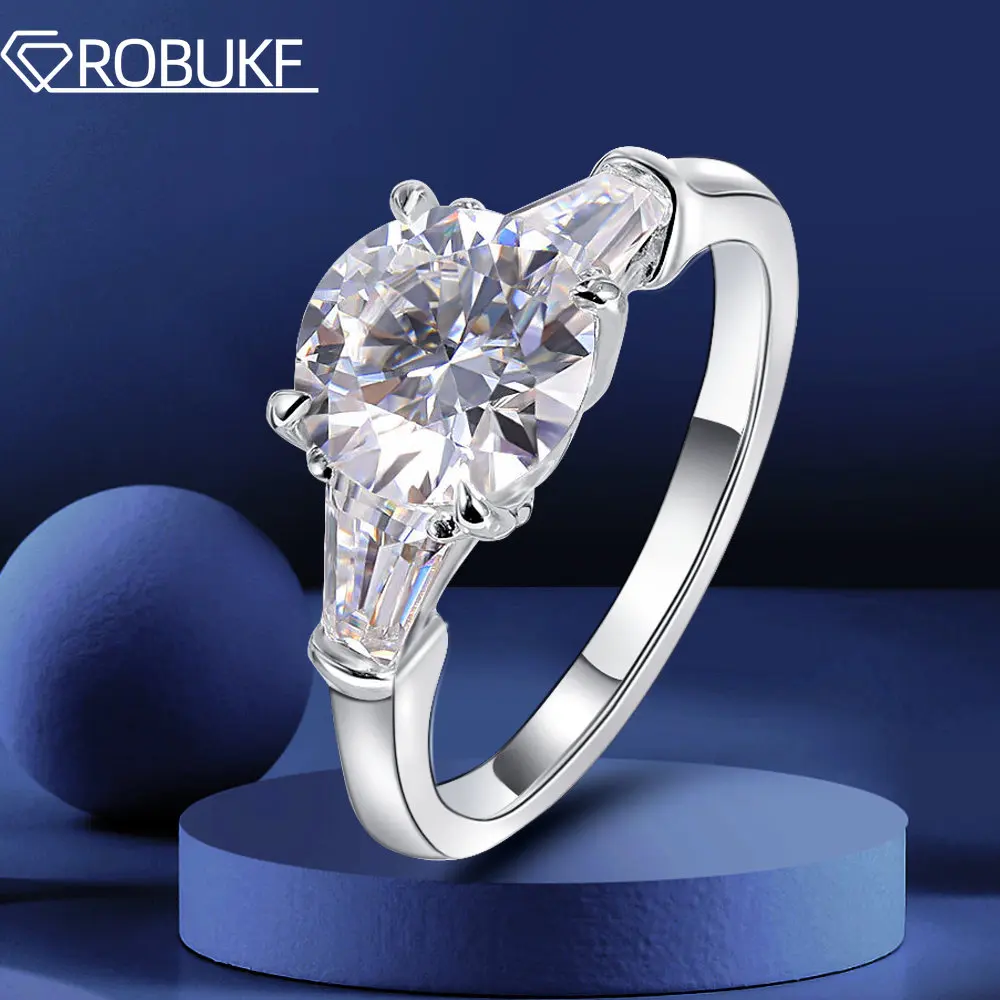This image is an advertisement for a company possibly called "ROBOKF" or "Robokov," with the brand name prominently displayed at the top in stylized lettering, accompanied by a logo symbolizing a diamond underneath. The primary focus is on an exquisitely designed diamond ring, presumably made of white gold or silver. The ring showcases a stunning, large central diamond, held by four clasps, likely weighing between three to six carats. Additional smaller diamonds inlaid in the clasps hint at intricate craftsmanship. The ring rests on an elegant blue, felt-like pedestal set against a darker blue background with subtle accents, adding depth to the presentation. Complementing the display, a blue sphere is positioned beside the ring, enhancing the visual appeal and sophistication of the advertisement.